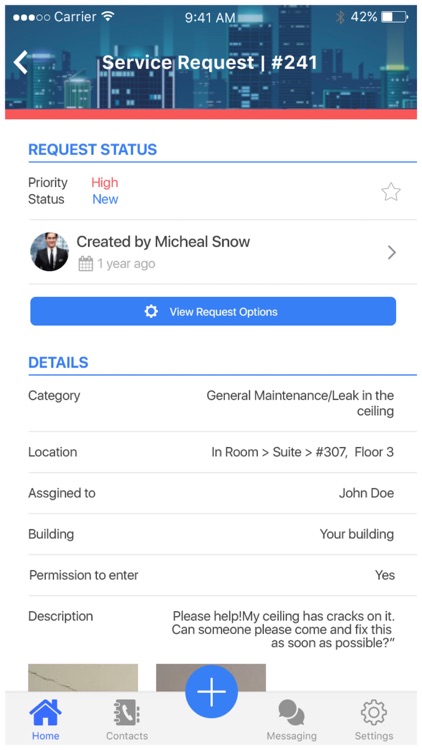The image displays a smartphone screen with several elements. At the top, the status bar shows cellular signal bars labeled "carrier" and Wi-Fi bars. The time displayed is 9:41 AM, and the battery is at 42%. Below this is a left arrow icon followed by "Service Request Number 241." The background features a nighttime cityscape with multiple high-rise buildings in various shades of blue. 

Below this section is a red strip, followed by a white background for the rest of the screen. In blue text, it reads "Request Status," followed by a blue line. Below this, in black text, it states "Priority: High" and "Status: New." To the right is an unticked star icon in a grey outline. 

A grey line separates the following section, which reads "Created by Michael Snow one year ago," with a right arrow icon on the right side. Below this is a large blue button spanning the width of the screen, with white text reading "View Request Options."

Further down, in blue text, it says "Details," accompanied by a blue line below it. It lists "Categories" on the left, and on the right it specifies "General Maintenance / Leak in the Ceiling." The text on the left reads "Location," and on the right "Room Suite Number 30743." The text on the left also indicates "Assigned to," with "John Doe" on the right. Additionally, it lists "Building" on the left, stating "Your Building," and has "Permission to Enter" on the left with "Yes" on the right.